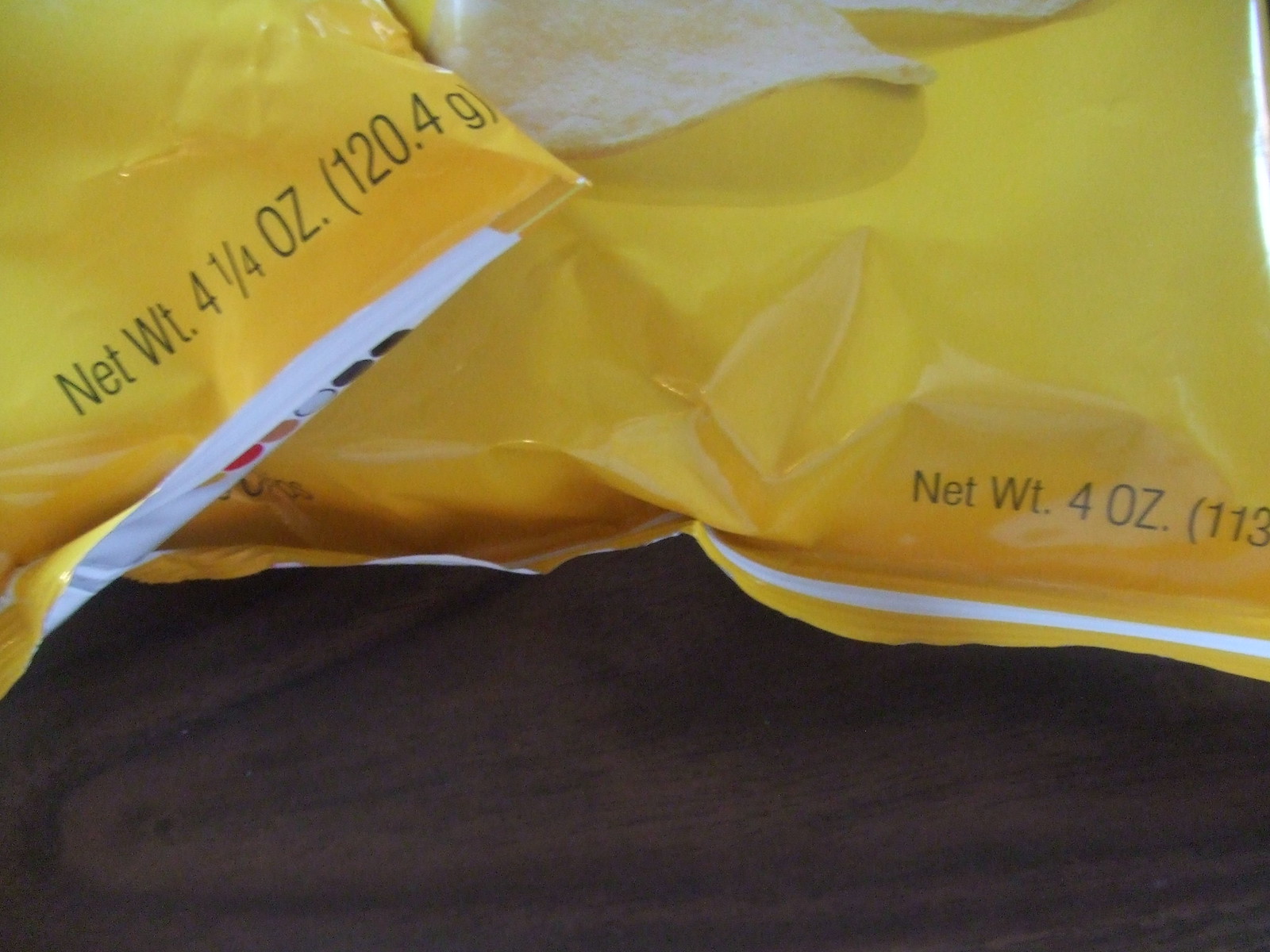In this image, two yellow bags of Frito-Lay plain potato chips are displayed on what seems to be a brown wooden table. The larger bag, prominently shown, features an illustration of a potato chip with visible text indicating a net weight of 4 ounces. The second bag, only partially visible with its bottom half obscured by the right corner of the larger bag, has a net weight of 4.25 ounces. The detailed visual of the potato chip on the bigger bag is clear, enhancing the branding and appearance of the packaging.